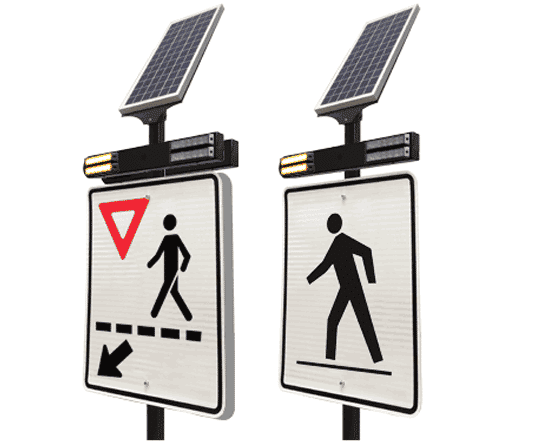This image depicts two vertical pedestrian crossing signs designed for street intersections. Each sign features a plain white background bordered in black. The left sign displays an upside-down red triangle in the upper left corner, signaling caution. Below it, there is a black stick figure of a person with a cane walking to the left, and beneath this figure is a downward-pointing black arrow towards the bottom left corner. The right sign shows a black pedestrian stick figure walking leftwards, with a horizontal black line beneath the figure indicating a crossing path. Both signs are mounted on a sturdy black metal pole. Atop each sign is an LED light bar intended to alert drivers and enhance visibility of the crossing area. Above each LED light bar is a rectangular solar panel, ensuring the signs remain powered and functional without the need to connect to the electrical grid. Together, these features create an effective combination of visual cues and advanced technological elements to promote pedestrian safety.